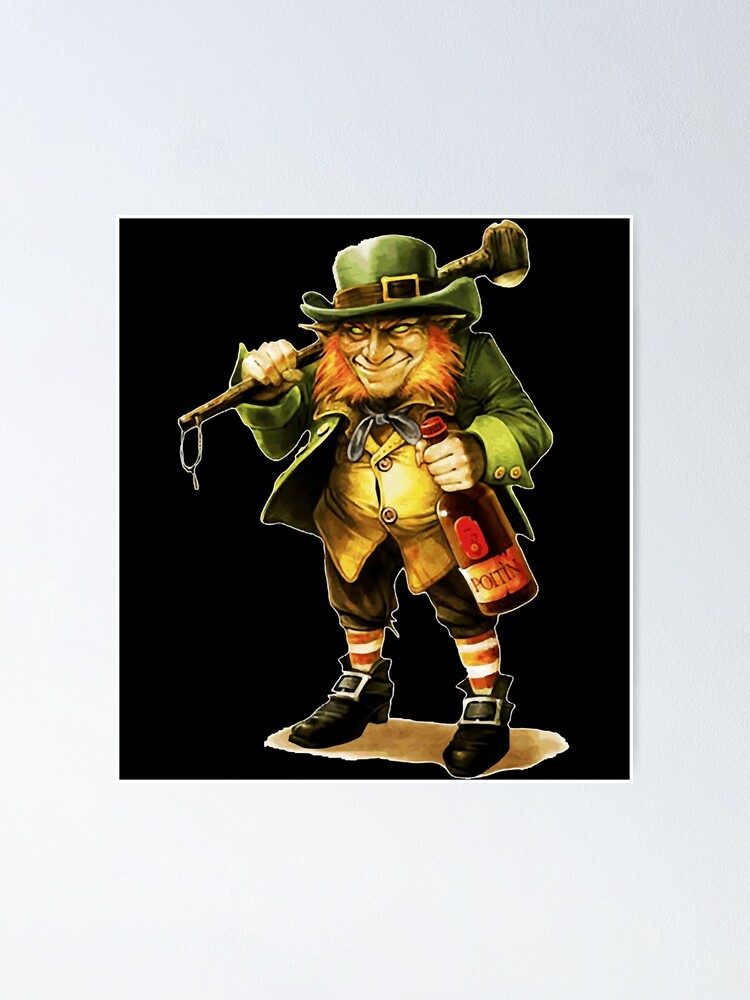This color photograph, framed in white with a stark black background, features a sinister-looking leprechaun. This malevolent figure boasts an orange beard and piercing greenish-yellow eyes that lack discernible pupils, adding to his eerie demeanor. His sharp, pointed chin and long, sinister nose are accentuated by a devilish smirk. Dressed in a dark green coat and matching top hat adorned with a black band and gold buckle, the leprechaun exudes a foreboding aura. His outfit includes a brown vest with buttons, short brown pants, and a yellowish shirt. Complementing his attire are black shoes with metal buckles and red and white striped socks. In his left hand, he clutches a black bottle with a red cap, labeled "POITIN"—a foreign word that resembles 'poison'. In his right hand, he holds a brown hammer resting behind his shoulder. The combination of his mischievous grin, the menacing items he holds, and his striking wardrobe all contribute to his overall menacing appearance.